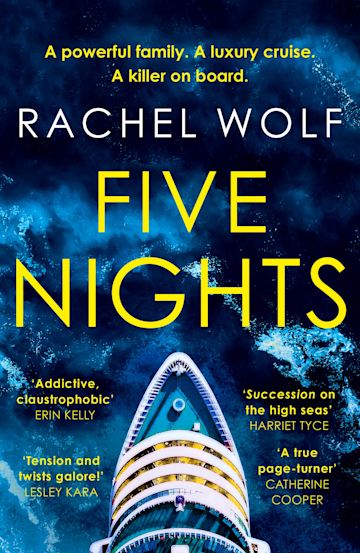The book cover features a dark blue ocean backdrop that lightens in the center, simulating the depths of the sea at night. Prominently displayed at the top, in yellow text, is the tagline: "A Powerful Family, A Luxury Cruise, A Killer on Board." Below this, in white text, is the author's name, Rachel Wolfe. The title of the book, "Five Nights," is presented in very large yellow text with "Five" and "Nights" each occupying their own line. The striking image at the bottom shows the front half of a cruise ship with a blue deck and white trim outline, splashing through the dark, cold waters. Surrounding the ship are multiple reviews in yellow text, including phrases such as "Addictive, Claustrophobic" by Erin Kelly, "Tension and Twists Galore" by Leslie Cara, "Succession on the High Seas" by Harriet Tice, and "A True Page-Turner" by Katherine Cooper.